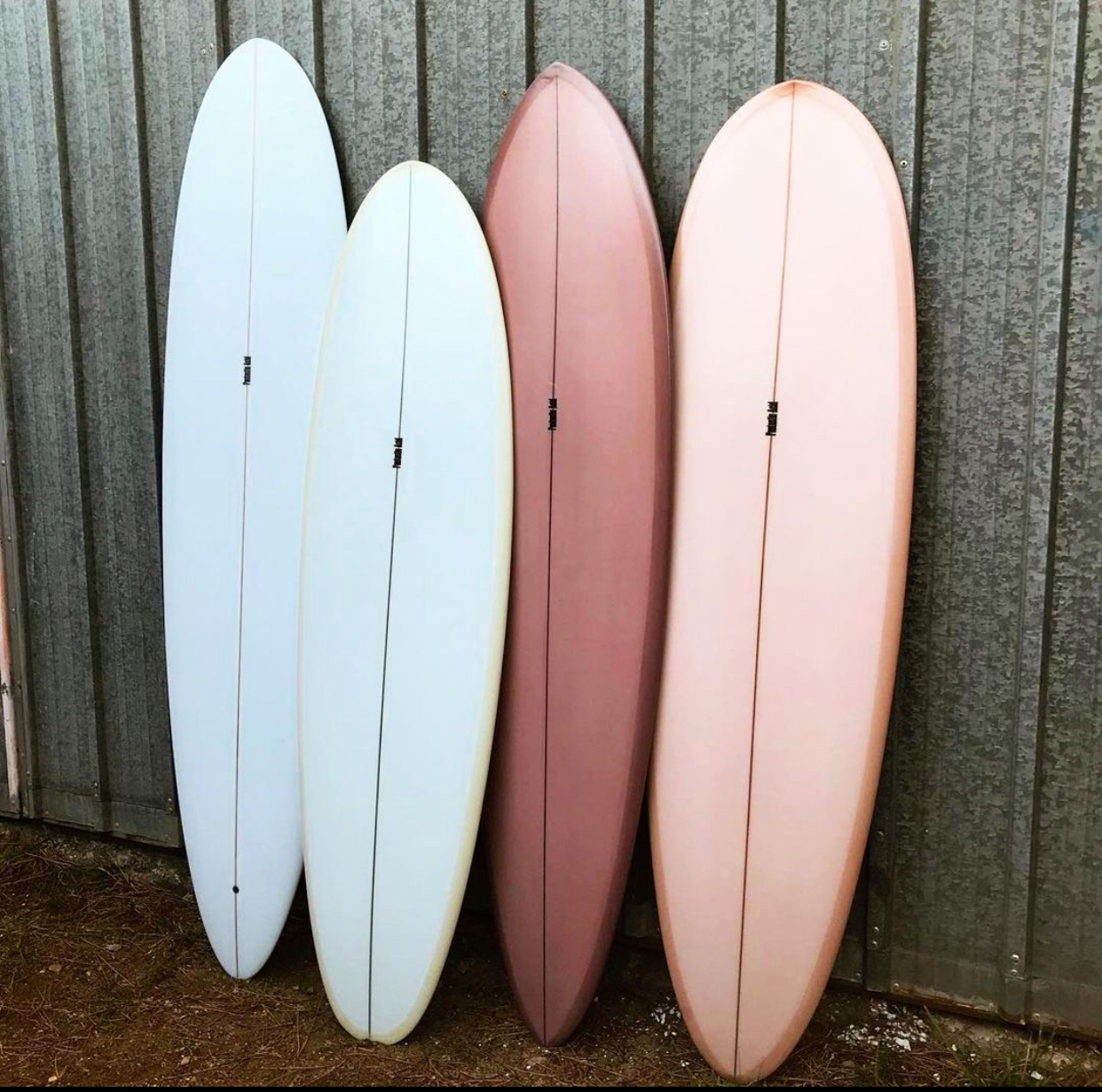This real-life photograph captures four surfboards leaning against a galvanized metal shed with a visibly weathered, rust-tinged bottom edge. The surfboards, each featuring a central crease with possible writing, display a variety of colors: the first on the left is a pastel blue, followed by a white one, then a deeper terracotta rose, and finally, a pastel peachy pink. Each board has a black object centered on its upper one-third. The ground beneath them reveals a natural setting characterized by patches of dirt, scattered pine needles, small twigs, and hints of white sand, alongside some sparse green grass. The metal surface behind the surfboards is detailed with vertical support shafts and rivets at the bottom.